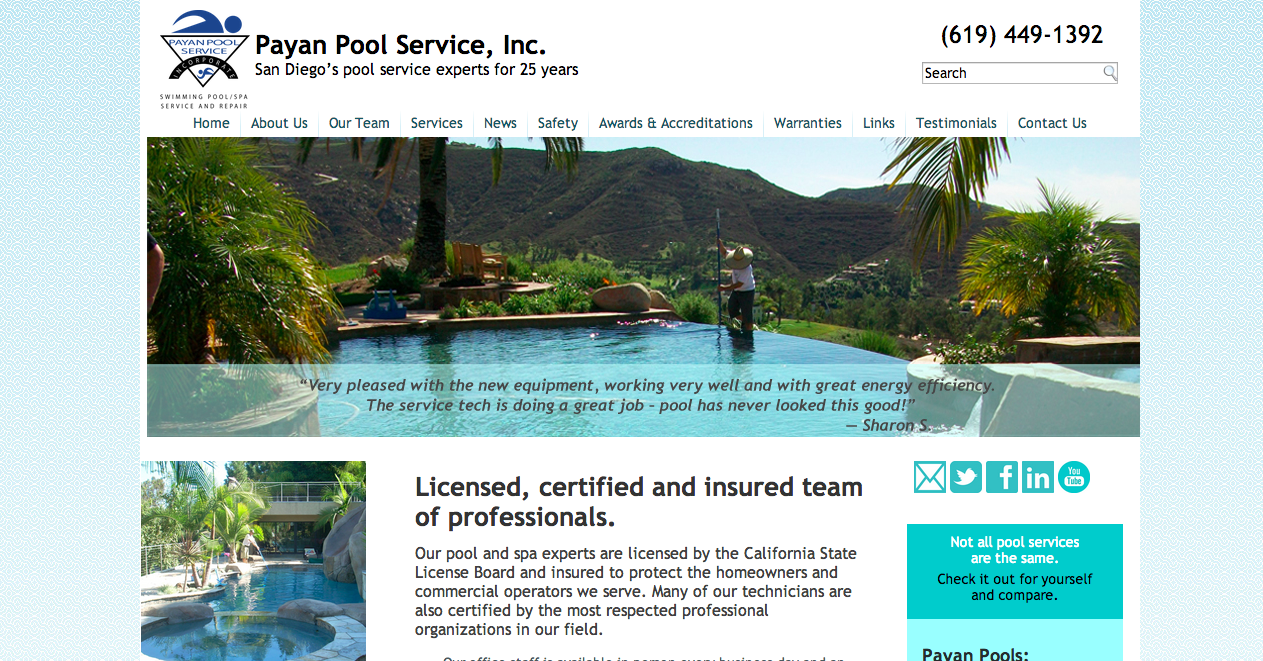This is a screenshot of the homepage for Payton Pool Service, Inc., showcasing their professional website layout. Their prominently displayed slogan, "San Diego's Pool Service Experts for 25 Years," reflects their extensive experience and commitment to quality. The company's logo, found on the left, features a triangle enclosing their name, and a swimmer above with one arm extended as if in mid-race, symbolizing their active and dynamic service.

To the right, there is a clearly visible phone number for easy contact, and just below it, a functional search bar for convenient website navigation. The main navigation menu stretches across the page, offering direct links to various sections: Home, About Us, Our Team, Services, News, Safety, Awards and Accreditations, Warranties, Links, Testimonials, and Contact Us.

Centrally positioned on the homepage is a striking banner featuring a lush landscape with a pristine pool as the focal point, where a man is actively cleaning it, highlighting their hands-on service. Below, on the bottom left, another image presents a serene pool and jacuzzi surrounded by palm trees, with city skyscrapers in the background, exemplifying their work in diverse environmental settings.

In the middle section, informative text emphasizes their licensed, certified, and insured status, assuring prospective clients of their professionalism and reliability. On the right, there are icons for social media sharing and updates, ensuring visitors can easily connect and stay informed about the latest from Payton Pool Service.